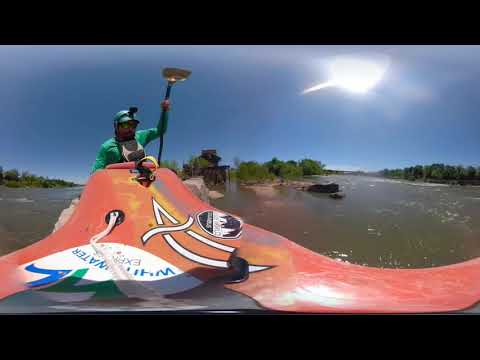In this vibrant fisheye photograph taken during the daytime, a man wearing a green long-sleeve shirt and a GoPro on his head is captured paddling a red canoe or kayak, adorned with white decals and a logo that includes the words "white water" in blue. The image, distorted from the wide-angle lens, features a scenic, brownish river or creek flanked by lush green trees on both sides. The bright blue sky above, possibly diffused by some clouds, adds a striking backdrop to this adventurous water scene. Subtle rock formations and patches of sand enhance the natural beauty of the surroundings.